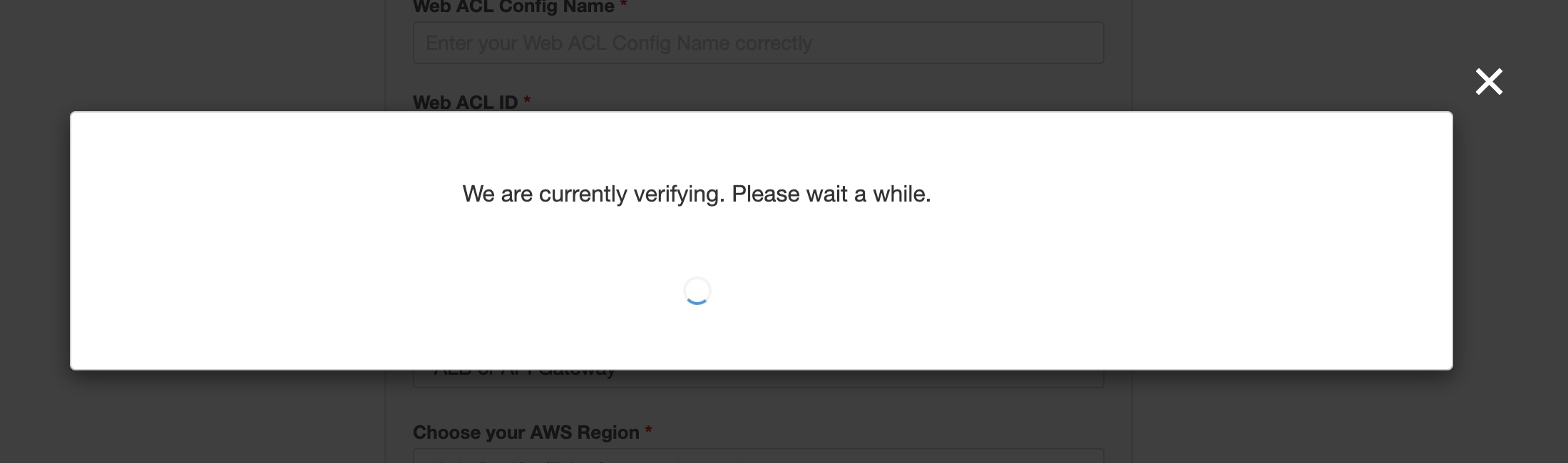A screenshot of a website displaying a pop-up window that grays out the background but still allows some visibility of the underlying content. The pop-up appears to be a form related to web ACL (Access Control List) configuration. The form fields include "Web ACL Configuration Name" with a red asterisk indicating a required field, and it prompts the user to enter the configuration name correctly. Another required field is labeled "Web ACL ID," also marked with a red asterisk, followed by an input box partially visible. Below it is the section "Choose your AWS Region," again with a red asterisk next to it, indicating it’s mandatory, with an input box beside it. 

At the top right corner of the pop-up, there's a white "X" inside a rectangle, allowing users to close the window. The pop-up displays a message, "We are currently verifying. Please wait a while," accompanied by a loading icon. The loading icon consists of a circle that is about 80% gray and 20% blue, suggesting that the blue segment is animated and represents the loading process.